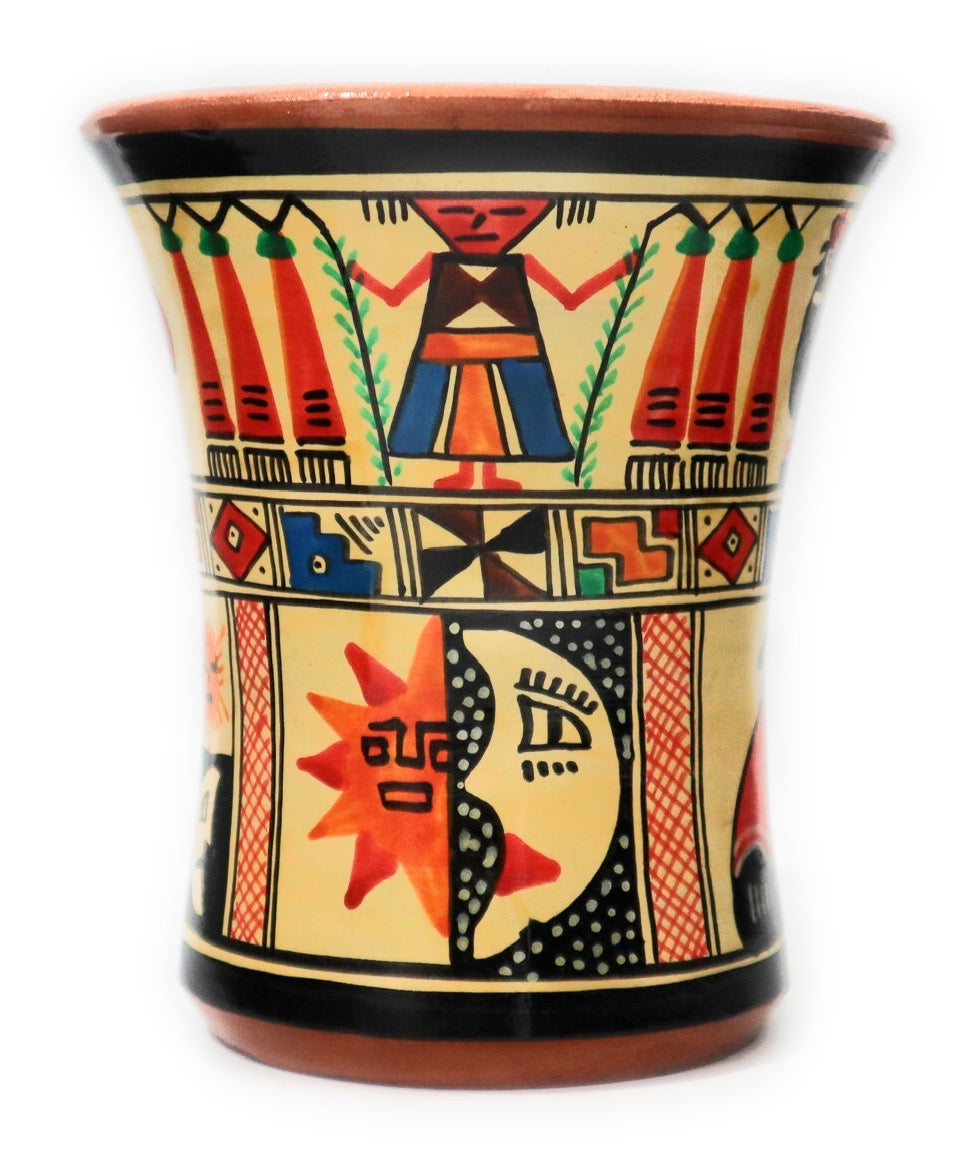This image showcases a beautifully crafted piece of terracotta pottery that has been glazed and intricately painted. The pottery sits against a pristine white background, with its edges on the left, right, and bottom artistically softened and blended into the surrounding white area using a subtle focus filter. The pot itself is shaped like a gently tapering cylinder that is wider at the top than at the base.

Adorning the surface of this pot is a mesmerizing design inspired by native or Aztec art, featuring prominently a depiction of the sun and moon near the bottom portion, with a figure of a man standing regally in the center of the top portion. The Native American-inspired motifs include a variety of geometric shapes and dots, all brilliantly rendered in a palette of vivid colors. The background of the design is a soft pastel yellow, providing a striking contrast to the bold hues of bright red, orange, blue, brown, and green that embellish the artwork.